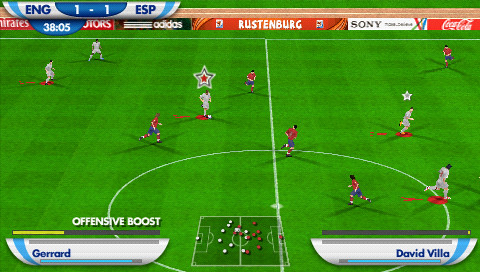The image depicts a vintage soccer video game characterized by its retro graphics. The vibrant green field stands out as two teams, one dressed in red and the other in white, compete intensely. The backdrop features classic advertisements from brands like Adidas, Sony, and Coca-Cola, adding an authentic touch of nostalgia. The scoreboard, situated on the left side of the screen, reveals a tied match between teams labeled ENG and ESP, each with one goal scored. A game timer accompanies the scoreboard, indicating the remaining match time. At the bottom of the screen, player icons hint at the interactive nature of the game, suggesting that it’s designed for user control and engagement.